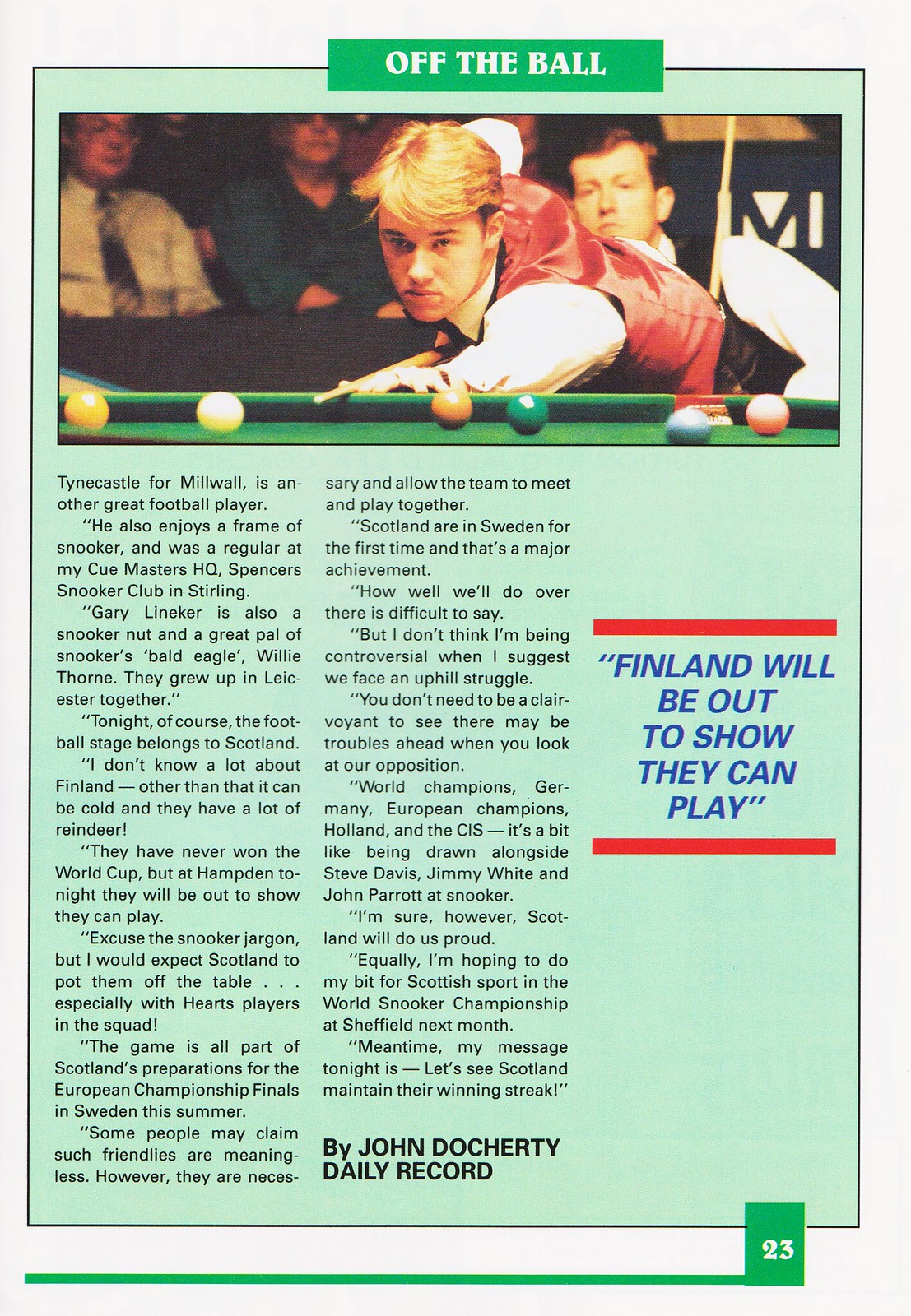The image, sourced from the Daily Record and credited to John Docherty, captures a dynamic moment of a man preparing to take a shot in a game of pool. The man, wearing a red vest and white shirt, is intently focused on the white cue ball, which is positioned in front of a colorful array of balls on the green felt table. A small green rectangle above the image contains the title "Off the Ball" in white letters, giving context to the pool scene. 

In the background, several spectators are visible, including a man in a white shirt with glasses, a woman in a dark blouse seated beside him, and another man in a black vest and white shirt holding an acoustic instrument. The scene appears lively with an audience engaging in the event. 

To the right of the image is an article, featuring paragraphs about various sports personalities and events. Among the details, it highlights Tyne Castle from Millwall, Gary Lineker's love for snooker, and mentions Spencer's Snooker Club in Sterling. The text emphasizes the night's focus on football, particularly Scotland's preparations for the European Championship finals in Sweden, and Finland's efforts to demonstrate their playing skills. The story concludes with a motivational message for the Scottish team and is signed off with "by John Docherty, Daily Record."